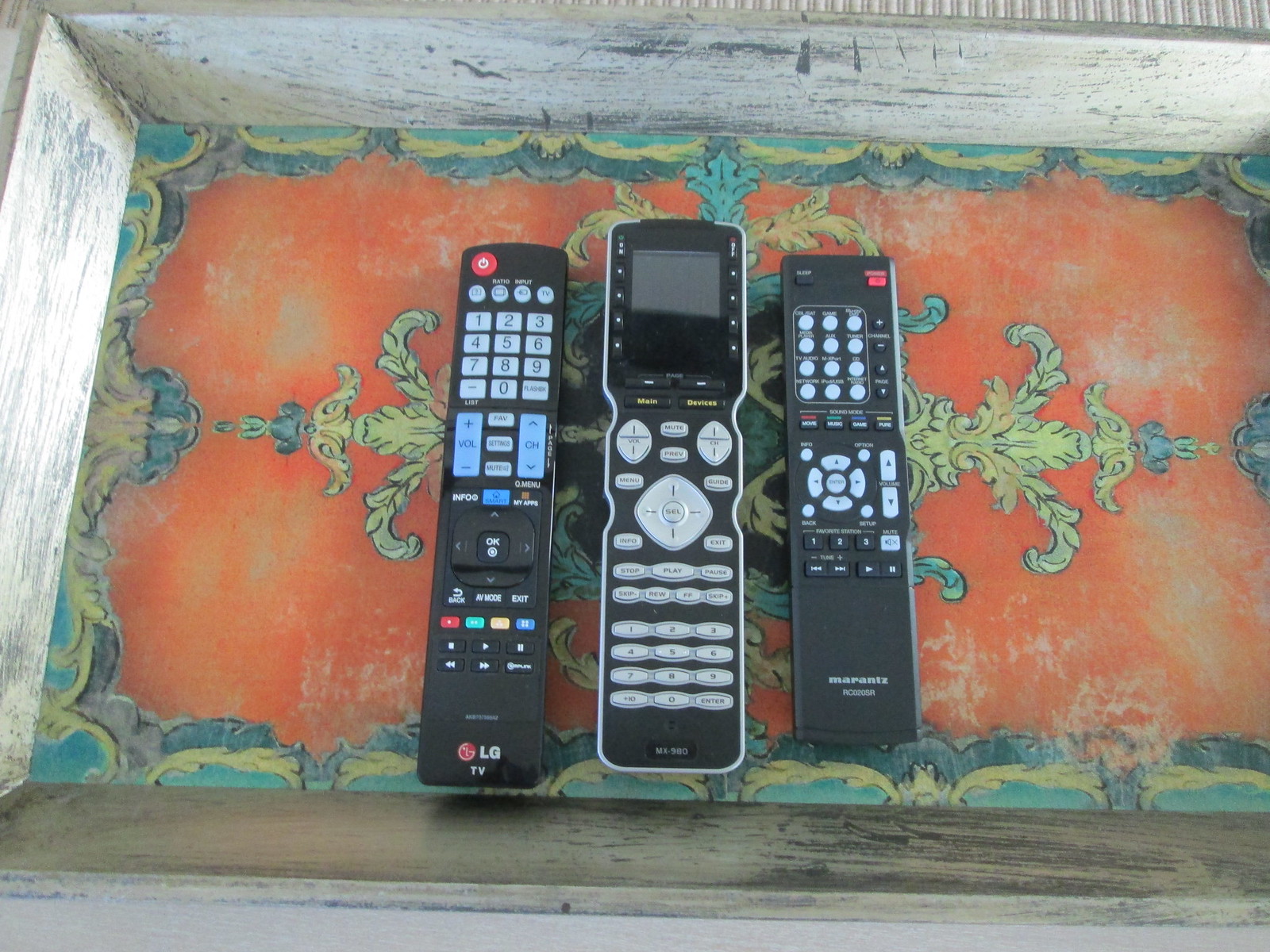The photograph features a weathered, vintage-style wooden tray lined with a faded red patterned paper, adorned with ornate green, yellow, and blue floral designs. Inside the tray, three black plastic TV remote controls are neatly placed side by side. The remote on the left bears the LG logo and includes a red power button among its numerous controls. The middle remote, marked with white text that reads "MI590" or "M something 980," also features an LCD screen. The rightmost remote is labeled with "Marantz." All three remotes are packed with an array of buttons, including volume, channel, number keys, and directional controls, indicating use with various entertainment devices. The rustic look of the tray, combined with the colorful yet faded interior pattern, creates a striking contrast with the modern appearance of the remotes.